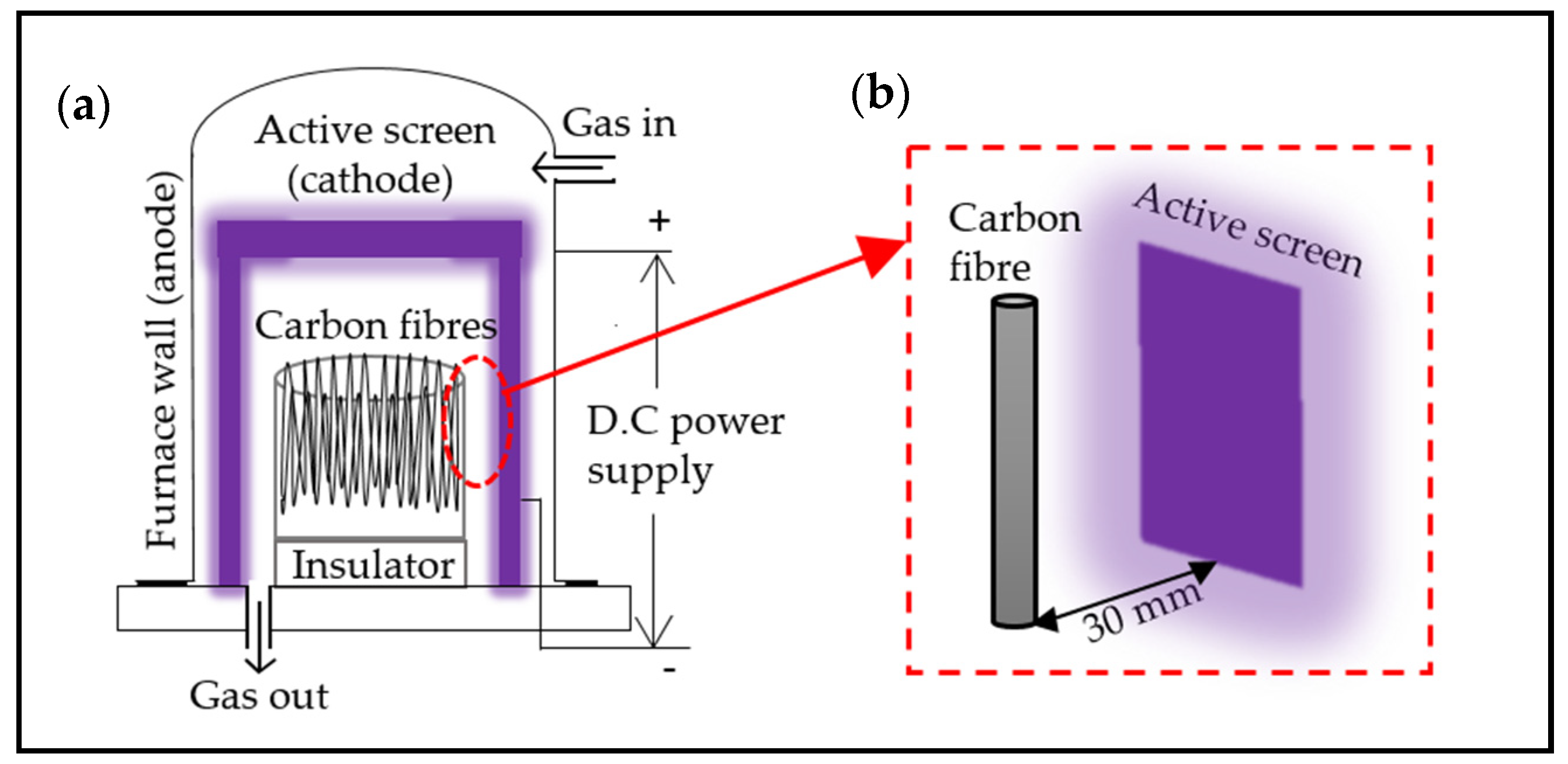The image depicts a detailed schematic diagram of a gas furnace system, presented in two parts: Diagram A and Diagram B, on a white background.

**Diagram A**:
- **Furnace Wall (Anode)**: On the left side, identified as the furnace wall, serving as the anode.
- **Active Screen Cathode**: Positioned centrally at the top.
- **Gas Inlet and Outlet**: Gas enters through an arrow marked 'gas in' on the right and exits via an arrow labeled 'gas out' on the left.
- **DC Power Supply**: Arrows indicating the flow of DC power, moving up and down below the gas paths.
- **Carbon Fibers and Insulators**: The central section below the active screen cathode is highlighted in a purple box, containing the carbon fibers depicted as black lines within a cylinder, with insulators below them.

**Diagram B**:
- **Zoomed-in View**: This part is a magnified segment of the area indicated by a red dotted oval in Diagram A.
- **Detail of Components**: Shows carbon fibers above a gray cylinder, with a rectangular purple block indicating the active screen.
- **Measurement**: The distance between the carbon fibers and the active screen is marked as 30 mm with arrows on either end.

Both diagrams emphasize the relative positioning and detailed structure of the furnace components, including the insulator, carbon fibers, and the pathways for gas and electrical input.